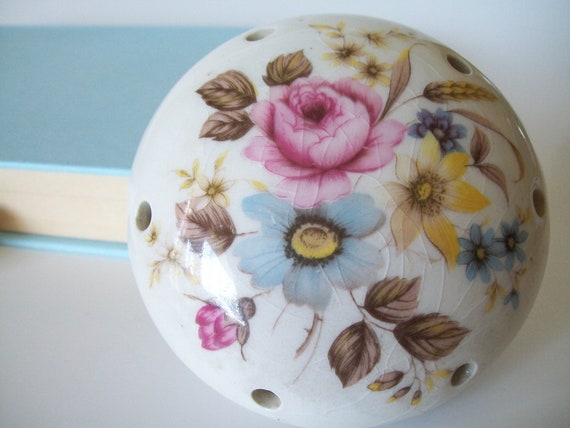The photograph features an antique ceramic sphere adorned with a detailed hand-painted floral design. The design includes a prominent red flower, a blue flower with a yellow center, and a yellow flower with a brown center, along with smaller blue and yellow blooms. Interspersed among the flowers are brown leaves, adding to the intricate pattern. The sphere exhibits signs of age, such as a crackle texture and minor cracks, indicating it may have been dropped but remains intact. Around its perimeter are six equidistant holes, reminiscent of those on a bowling ball, though not arranged in the same formation. The object stands against a slightly blue background, possibly a wall or a closed book with a blue cover. The ceramic item may have originally served as a vase or a decorative piece, and there's a suggestion that it could feature a removable lid, although this isn't clear in the image.